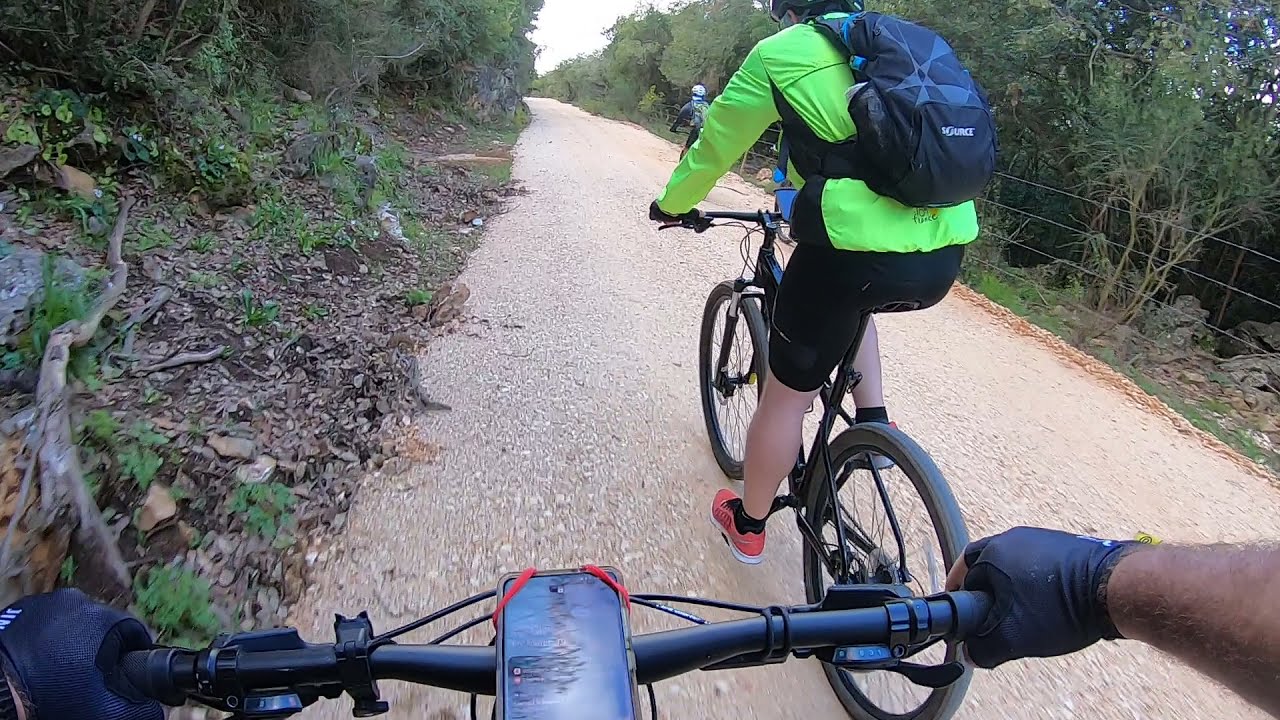This first-person view image captures a daytime mountain biking scene on a light tan, rocky, gravel path flanked by lush forest. The photo, taken from over the handlebars of a biker wearing black gloves and holding a phone-mounted handlebars, prominently features three cyclists. The closest rider, directly in front, is seen from behind, pedaling forward on a black-framed bike. This rider is wearing a neon green jacket, black shorts, a blue backpack, and sneakers. About 20 feet ahead is another cyclist clad in a black jacket and a white helmet, cruising farther along the path. Both sides of the trail are densely populated with trees, and to the right, a barbed wire fence or high-tension wires mark the boundary. The scene is well-lit by daylight, with a glimpse of the bright sky above.